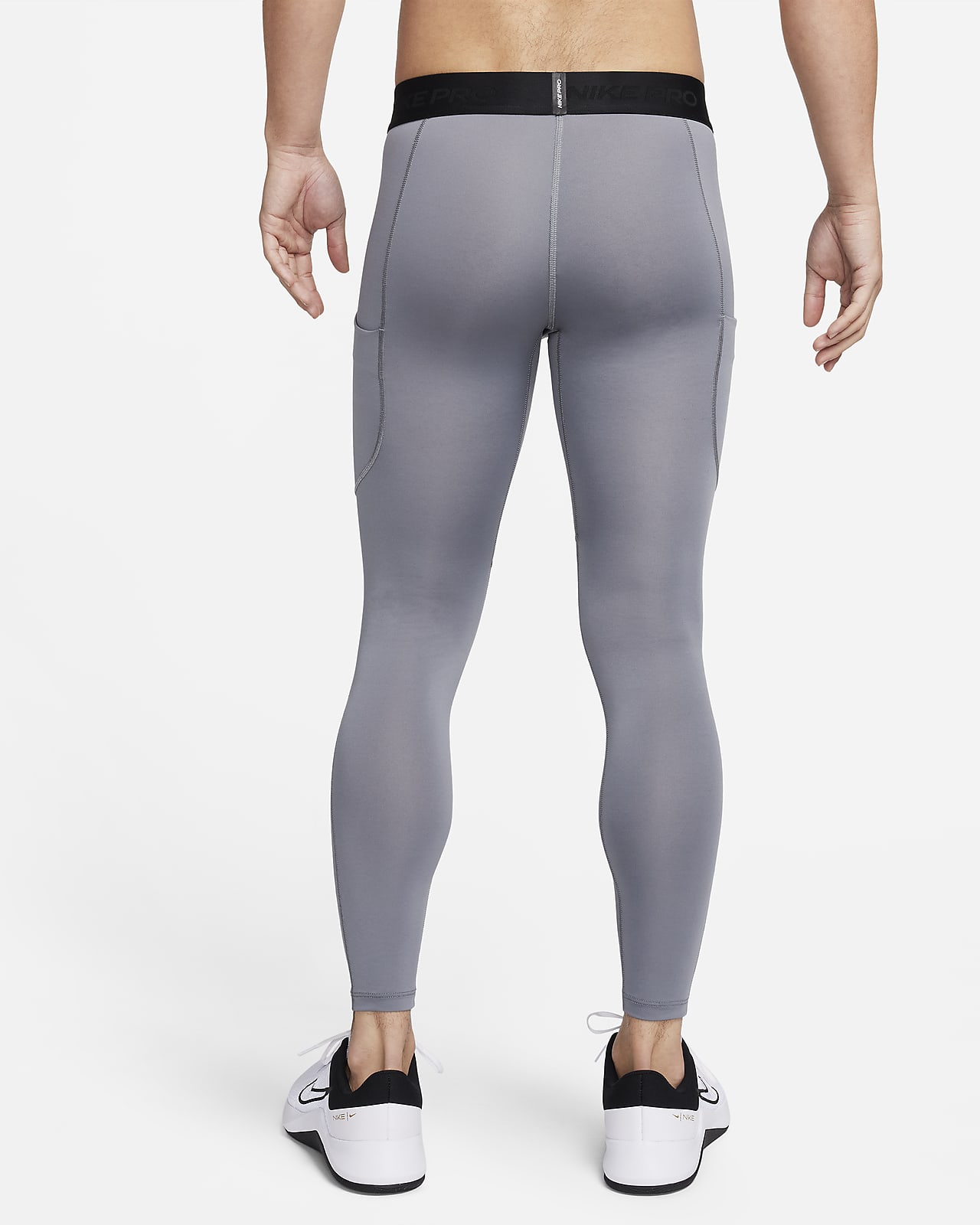This up-close image showcases the lower back down to the ankles of a well-built, muscular Caucasian man. His arms hang relaxed by his sides, and his upper body is unclothed, revealing a portion of his bare lower back. He is wearing tight-fitting, light gray spandex pants with a black elastic waistband. The pants are highly form-fitting, emphasizing his athletic build and muscular legs, with seam details running down the center and sides, as well as small pocket slits. The pants extend down to his ankles, where he is seen wearing white tennis shoes with a black collar and a visible black Nike swoosh on the side. The background of the image is a very light gray, adding contrast to the subject’s athletic attire.